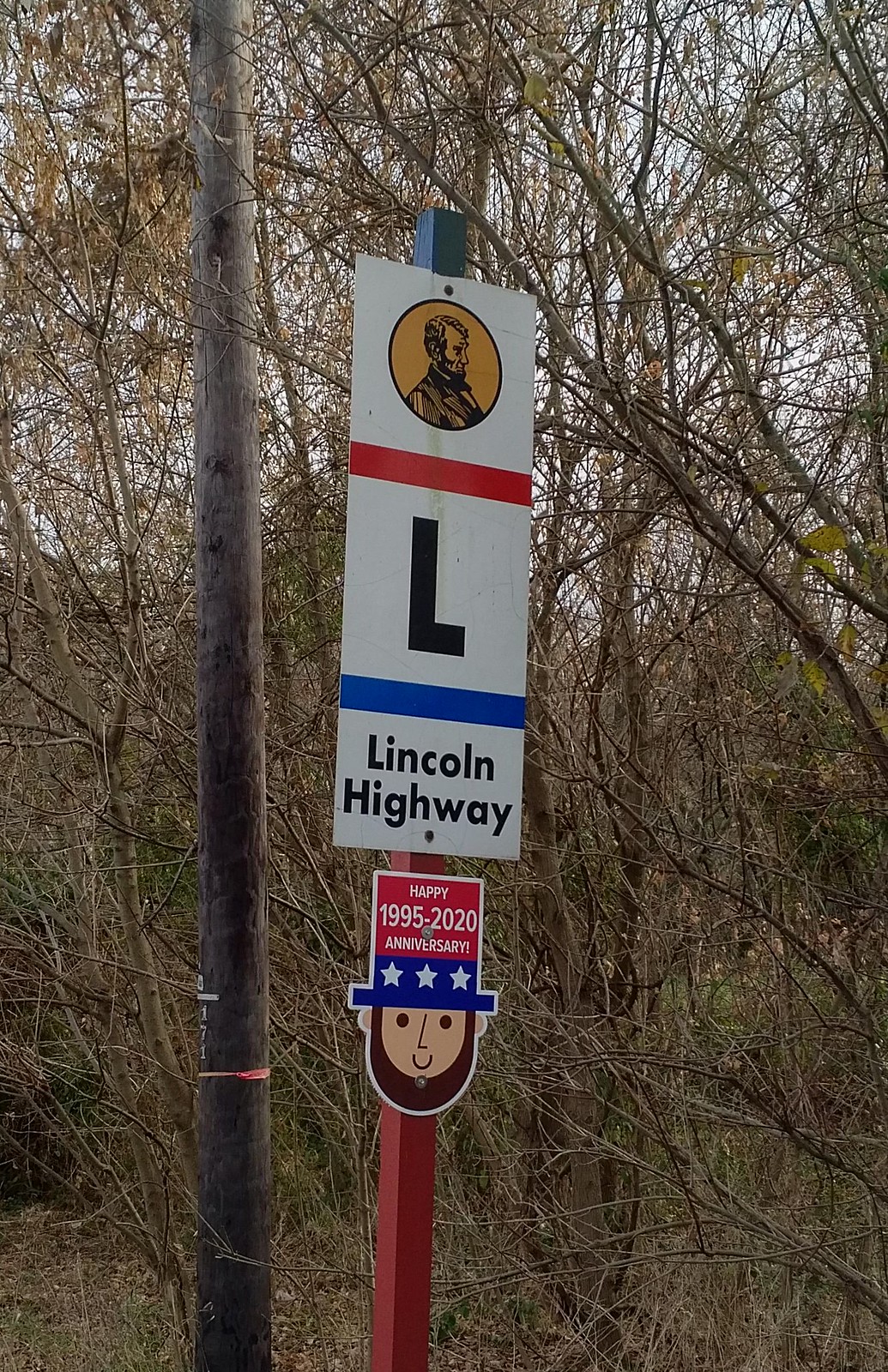The image is a vertically oriented outdoor color photograph showcasing an eye-catching signpost. The signpost begins with a square post that transitions from red at the bottom to blue at the top. Attached to the post are two signs. The uppermost sign features a photograph of a Lincoln penny, adorned with a horizontal red stripe, a large black letter 'L', a blue horizontal stripe, and the words "Lincoln Highway" in black text. Below this sign, there is a uniquely shaped sign resembling President Abraham Lincoln, complete with a beard. His top hat is festively decorated in red, white, and blue with stars, and it reads "Happy 1995 to 2020 Anniversary." The bottom portion of the post is lit up, possibly illuminating Lincoln's smiling face. The background includes telephone poles, a tree line, sparse foliage, and a cloudy white sky, indicating an overcast day. Twigs and brush are visible at the base of the post, adding to the natural roadside setting.